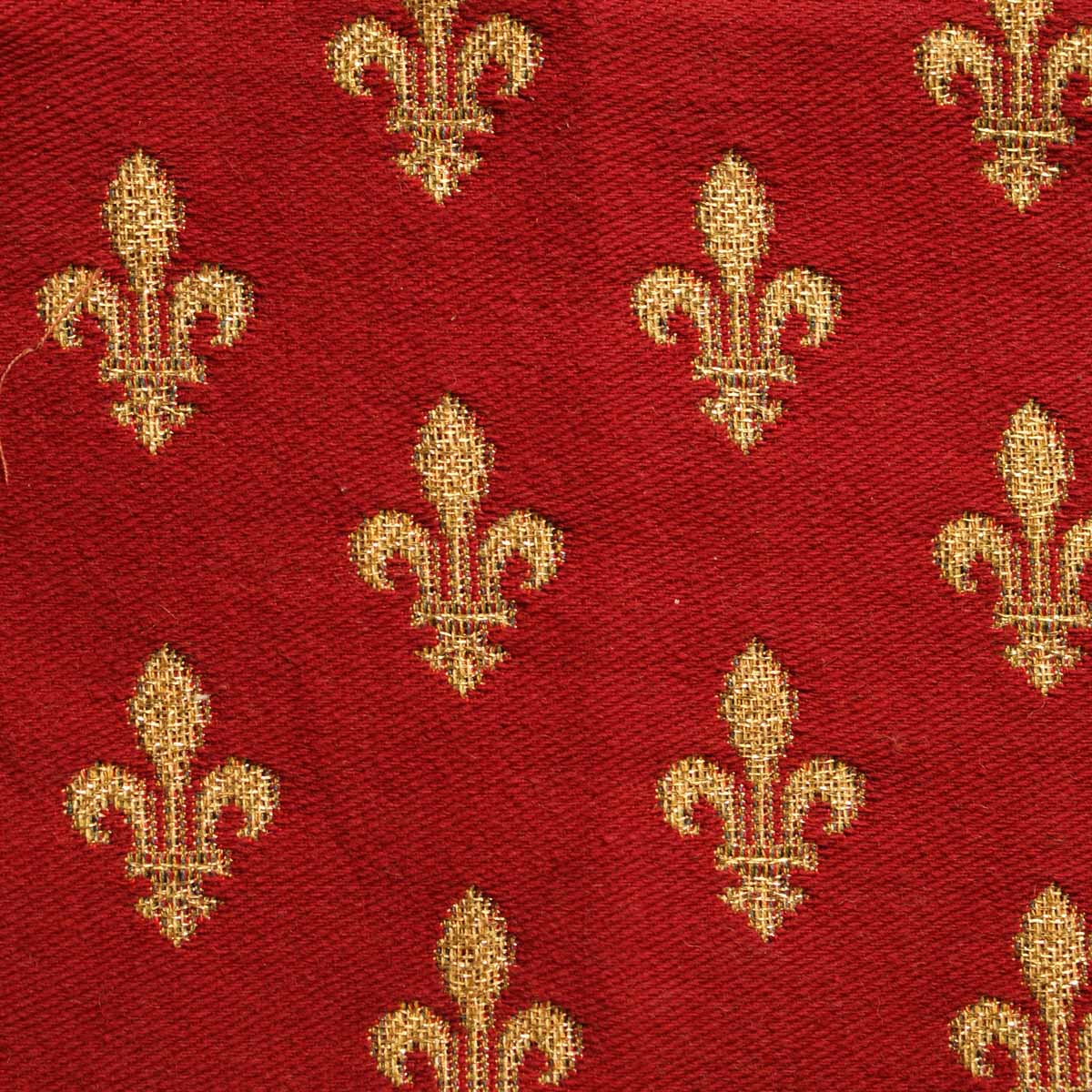The image is a square textile featuring a deep red background. The red hue transitions from darker on the left to lighter on the right, showcasing intricate stitching throughout. Spread across the fabric are patterned decorative symbols in gold, each composed of a central tall structure resembling a spoon, with curved elements on either side reminiscent of leaves. The base of each symbol features an upside-down crown-like crest. These symbols, described as yellow crests or decorative elements, are spaced apart in a staggered arrangement, ensuring they are neither vertically nor horizontally aligned. Fine embroidery details embellish the entire piece, enhancing its intricate and elaborate appearance.